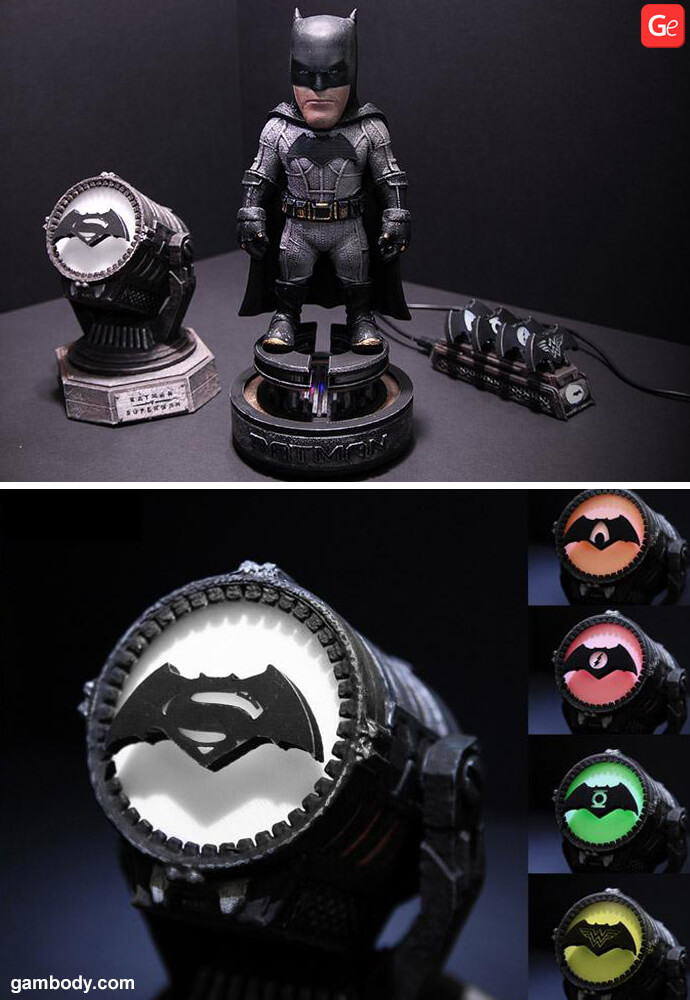The image is comprised of two stacked photos, each capturing distinctive elements of a Batman-themed collection. In the top picture, a Batman figurine stands prominently on a small round display pedestal, facing the camera. He is adorned in a classic all-black Batman suit with a cape, featuring the iconic Bat symbol on his chest. The head of the figurine appears notably large in proportion to its body. To the left of Batman, the metallic gray base of the Bat-Signal is visible, with a black Bat-Signal device that projects the bat icon into the sky. To the right of Batman, a set of four batarangs is visible, each contained within a pack. The upper right corner of this picture also includes a red box with the white letters "GE." The bottom picture provides a close-up view of the Bat-Signal, displaying a prominent black Bat symbol. To the right, a range of alternative Bat-Signal styles is showcased, including options with lights in orange, red, green, and yellow. The image's lower corner includes the branding "GAMBODY.COM" in white lettering.